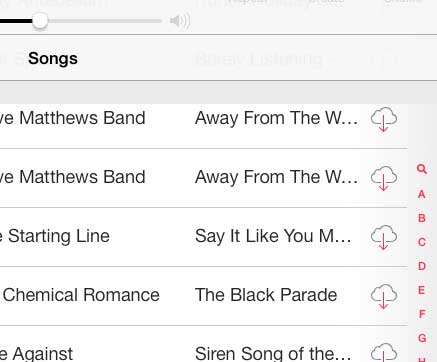This is a zoomed-in screenshot capturing a segment of a music library app that bears a resemblance to the classic interface of iTunes. At the very top of the screenshot, the right side of a sound bar is visible with the volume level partially turned up, but not at maximum. In bold black text at the top left corner, the word "Songs" is prominently displayed. 

Beneath this heading, portions of five different bands along with their respective song titles can be seen. The first entry is for "Dave Matthews Band," though only "ve Matthews Band" is visible. The song title associated with this band is truncated to "Away From the W...". The second line mirrors the first, showing another entry for "Dave Matthews Band," again with the song title partially visible as "Away From the W...".

The third line presents a partial band name, "The Starting Line," with the song title cut off to "Say It Like You M...". 

The fourth line features "My Chemical Romance," completely visible, alongside the full song title "The Black Parade."

On the fifth and final line, only the letter "E" followed by a space is visible, likely part of the band name "Rise Against." The song title associated with this last entry is not entirely clear in the screenshot.